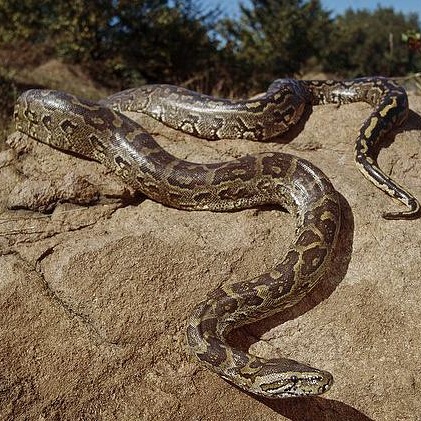This is a detailed photo of a medium-sized, snake with a thick body, resting on a brown rock. The snake features a color pattern of brown and dark greenish-brown with distinctive spots, giving it a slightly camouflaged look against the similarly colored rock. The snake is coiled with its head visible at the bottom right of the image, one eye peeking out, and its body winding through the center and upper part of the image, ending with its tail waving at the top right. The background reveals green bushes and trees, with a glimpse of blue skies, indicating it's a sunny day. This close-up captures the essence of this potentially intimidating snake in its natural, outdoor habitat.